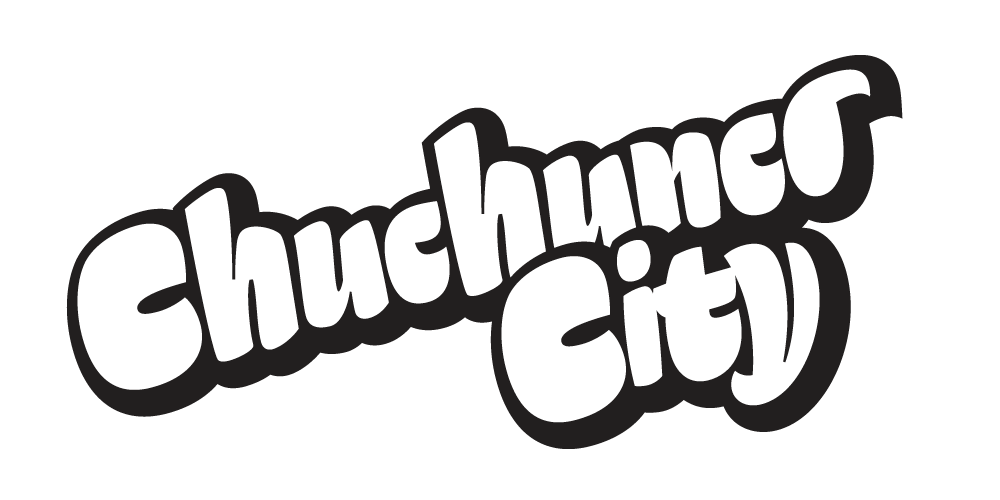The image depicts a purely textual graphic, potentially a logo, featuring the name "Chuchuner City." The design showcases thick, bubble-style letters, rendered in a three-dimensional manner with white interiors and black borders, creating a bold and eye-catching effect. The text is angled, starting from the lower left and ascending to the upper right, with "Chuchuner" positioned prominently above and slightly behind the word "City." The word "City" is easier to read and is offset to the right of "Chuchuner," overlapping it slightly. The entire composition stands out starkly against a plain white background, emphasizing its clean, graffiti-inspired style.